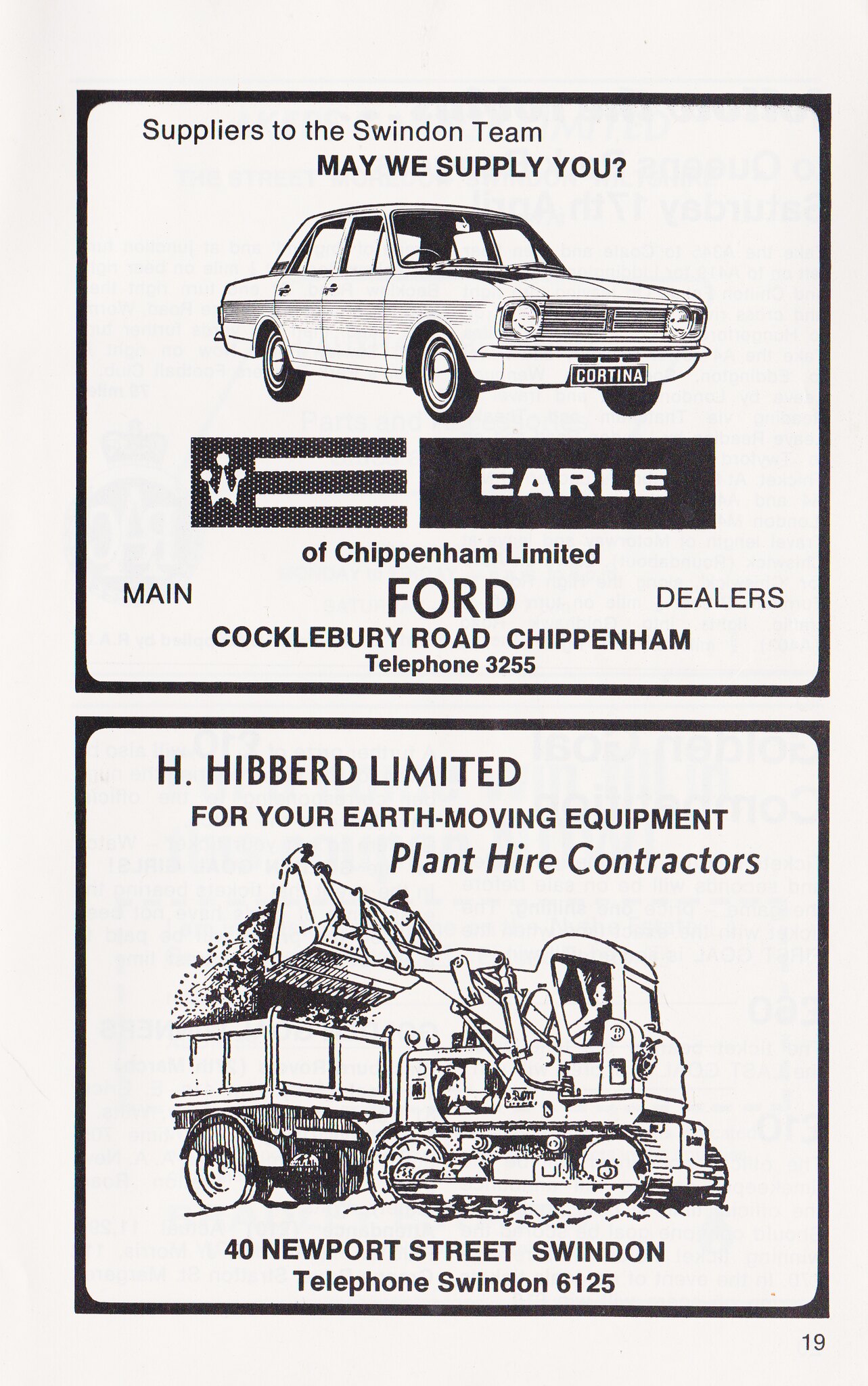The image features a page from a magazine showcasing two vintage advertisements stacked vertically. The top advertisement, bordered with a thin black outline, is a simple black and white design promoting "Suppliers to the Swindon Team." In bold letters, it asks, "May we supply you?" Below this, an illustration of an old car appears, with "Cortina" displayed on the license plate. Further down, it reads "Earle of Chippenham Limited," denoting the main Ford dealers located at Cocklebury Road, Chippenham. The contact number provided is telephone 3255. 

The second advertisement below is for "H. Hibbard Limited," highlighting their services in earth-moving equipment and plant hire contracting. This ad features an illustration of machinery dumping rocks into the back of a wagon. The company's address is listed as 40 Newport Street, Swindon, with the contact number being Swindon 6125. 

Both ads likely served as sponsors or local business promotions, reflecting a bygone era through their simple, illustrative style and detailed contact information.